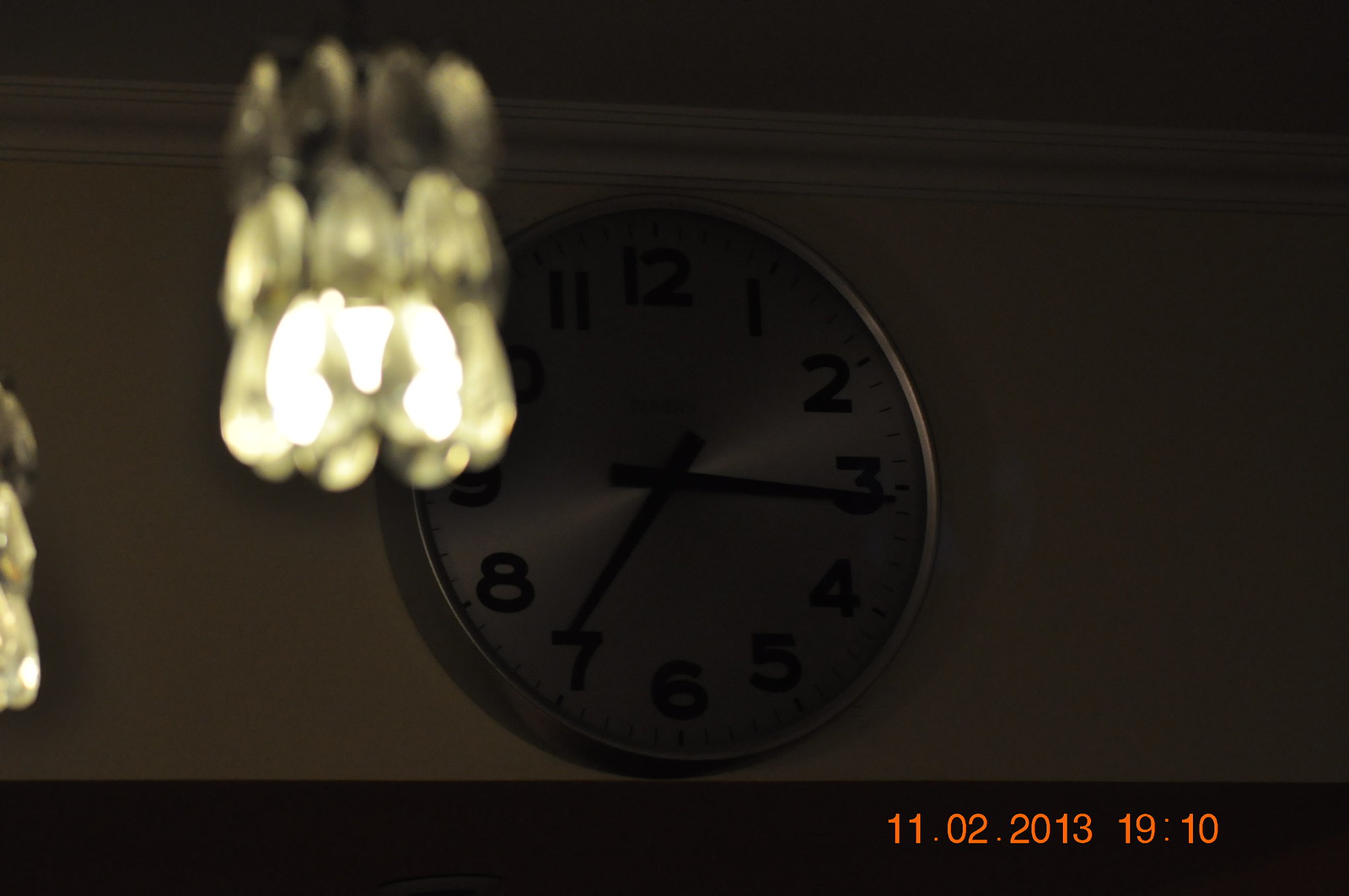In this dimly lit, blurry color snapshot dated November 2nd, 2013 at 19:10 (7:10 PM), a simple wall-mounted clock with a stainless steel or brushed frame and a white or possibly gray face is seen high up near the crown molding. The clock features black numbers and black hour and minute hands, though the second hand and brand name inscribed above the hands remain indiscernible due to the low light. The lower part of the image has a horizontal orange-glowing date and time stamp. To the left of the clock, a three-tiered light fixture resembling a chandelier with seashell or crystal-like shapes is visible, its tiers forming a cylindrical shape. Another portion of a similar light fixture is just barely cropped at the very left edge of the photo. The room itself appears deeply shadowed, casting a purplish hue over the scene.